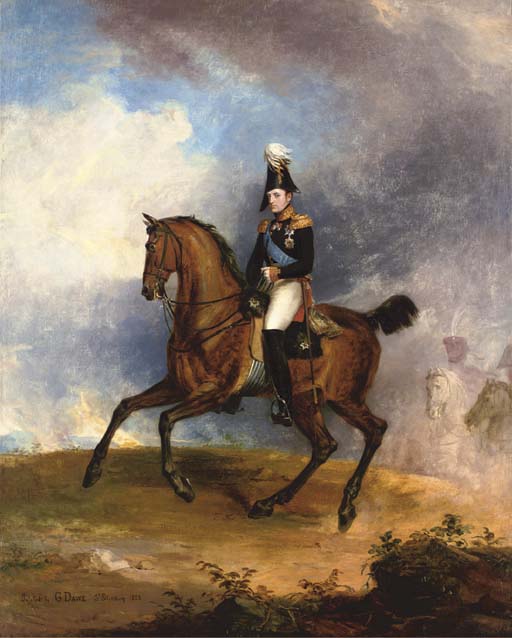This detailed oil painting depicts a military figure resembling Napoleon on a galloping brown horse. The man, appearing to be in his thirties, is attired in a formal black uniform, adorned with gold shoulder pads, a blue sash, and multiple medals on his chest. He is also wearing white breeches, black riding boots, and a distinctive black military hat with a fluffy white plume on the top. The horse, captured in mid-motion, is moving from right to left across a yellowish-green and brown ground. The background features a dramatic blue sky filled with heavy white and dark clouds. Additional elements include faint images of other horses and a bearded man partially obscured by clouds or smoke to the right side of the painting. The artist's signature is visible in the bottom left corner, indicating the portrait orientation of the work.